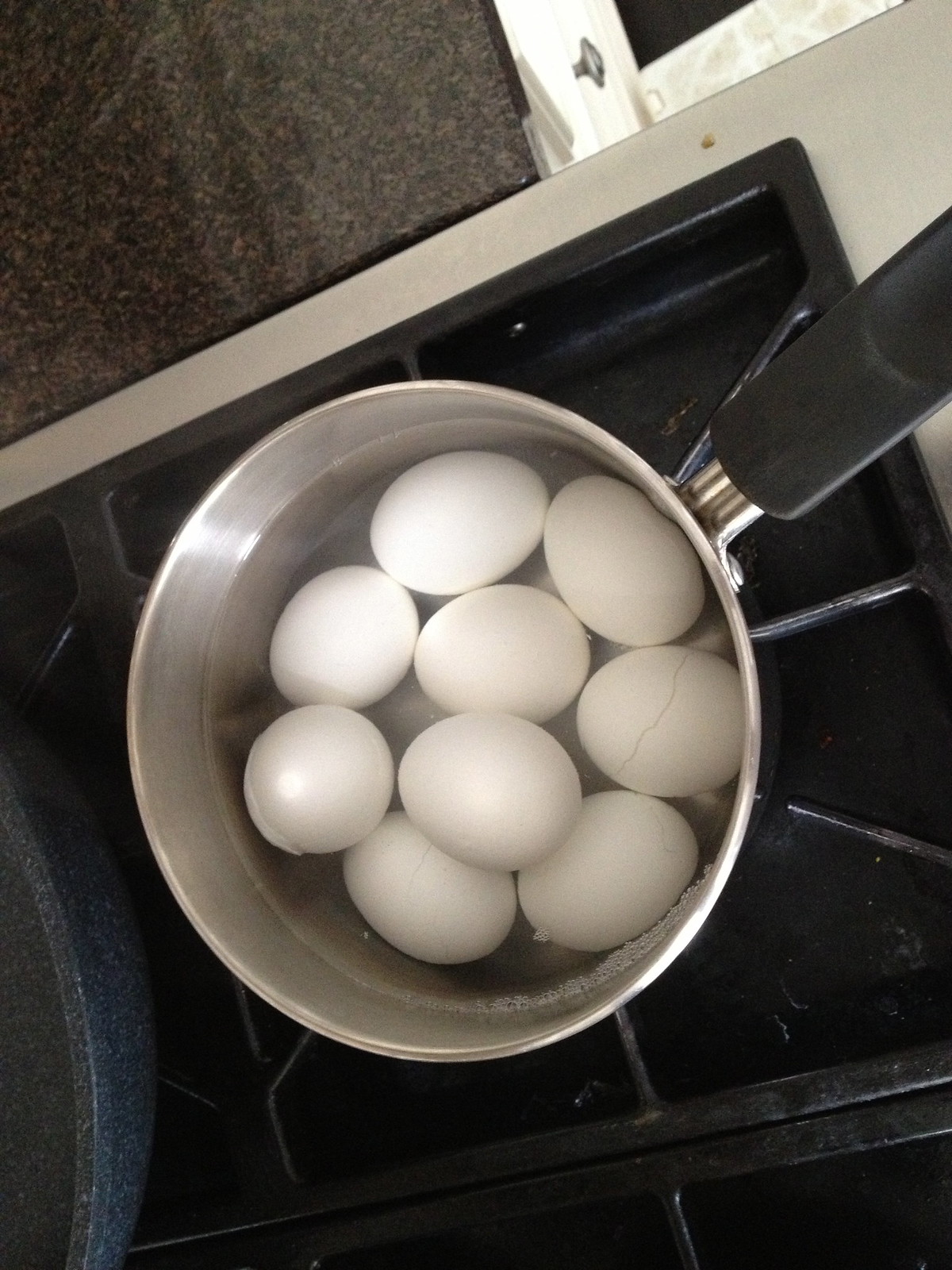In a cozy kitchen setting, an overhead image captures a stainless steel pot with a black handle sitting on a black gas stove. The pot is filled with water and contains nine white eggs, presumably being hard-boiled. The water shows signs of recent boiling, evidenced by a few small bubbles and a slight cooling phase. Notably, two of the eggs have cracks, with one significantly cracked and the other slightly so, indicating they have indeed been boiling. Positioned nearby, a dark blue pot with a gray nonstick interior rests on the stove. The stove's surface has metal trim around the burners, and the surrounding counter space has a tan finish. Also visible is the black laminate flooring beneath, providing a subtle contrast to the kitchen's neutral hues.